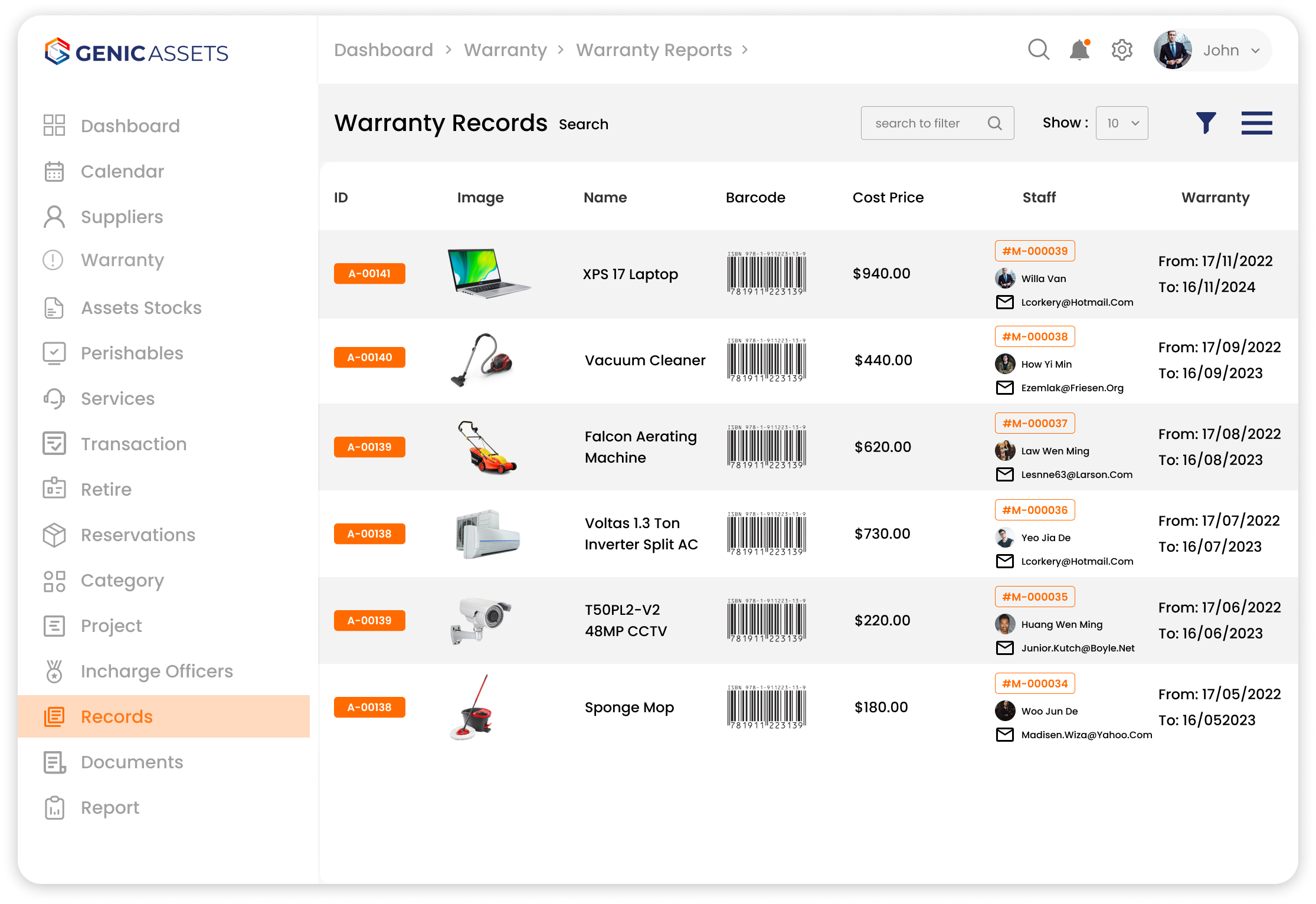In a slightly rectangular image oriented horizontally, the scene depicts a person engaged in online shopping through either a mobile app or website. The layout is divided into two main sections: a left-side column and a main body on the right.

The left column is headed with "Genic Assets," accompanied by an unidentified icon, presumably the company logo. Beneath this header, a list of functionalities runs down the length of the column in gray text. The options listed include: Dashboard, Calendar, Suppliers, Warranty, Asset Stocks, Perishables, Services, Transaction, Retire, Reservations, Category, Project, In-Charge Officers, Records, Documents, and Report. Notably, the "Records" option is highlighted with an orange box and displayed in orange text, indicating it is currently selected.

In the main body of the image, the interface suggests that the user is browsing items possibly related to warranty management. The interface displays headings such as Dashboard, Warranty, Warranty Reports, and Warranty Records Search. Below these headings, a list of various products is visible alongside images, including items like a laptop, lawnmower, vacuum cleaner, and camera. Each product entry includes accompanying details such as prices and dates, helping the user make informed decisions.